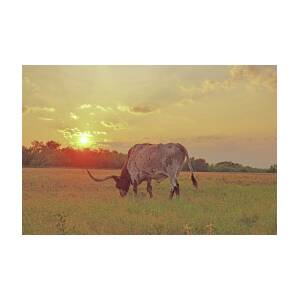In this landscape-oriented painting, a longhorn steer is the central subject, elegantly grazing in a lush, green pasture at sunset. The steer, with its prominent curved horns, stands facing left, its head bowed to munch on the grass. It has a distinctive appearance: a black head, a white and cream-colored body, a black-tipped tail, and black feet. The serene scene is bathed in the warm hues of the setting sun, which casts a purplish-orange glow across the sky. The sun is nestled near the horizon to the left, partially obscured by a distant tree line that stretches horizontally across the landscape. Clouds gather in the upper right corner of the image, adding to the tranquil atmosphere. The rich tapestry of dark green trees in the background contrasts beautifully with the vibrant field in the foreground, creating a harmonious balance between the natural elements.